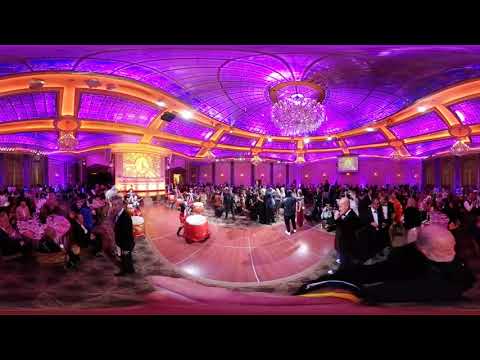This is a panoramic 360-degree image of an ornate ballroom, characterized by its expansive and decorative design. The room features a large wooden dance floor in the center, noticeable for its glossy finish that reflects the bright lights hanging above. Surrounding the dance floor are sections of carpeted areas where many people are seated, while others stand and engage in conversations. 

A standout feature of the ballroom is its vividly designed ceiling, shimmering in metallic purple tones and adorned with an intricate orangish-yellow pattern reminiscent of railroad tracks. Dominating the center of the ceiling is a radiant crystal chandelier, casting a brilliant light that enhances the room’s elegance. 

The ballroom’s walls and lighting enhance the space's festive ambiance with their bright and vivid purple glow. In one corner, groups of elegantly dressed people are engaged in lively discussion, and behind them, a large golden image is projected onto a screen. Both men in tuxedos and women in splendid dresses populate the room, adding to the overall grandeur and celebratory atmosphere.